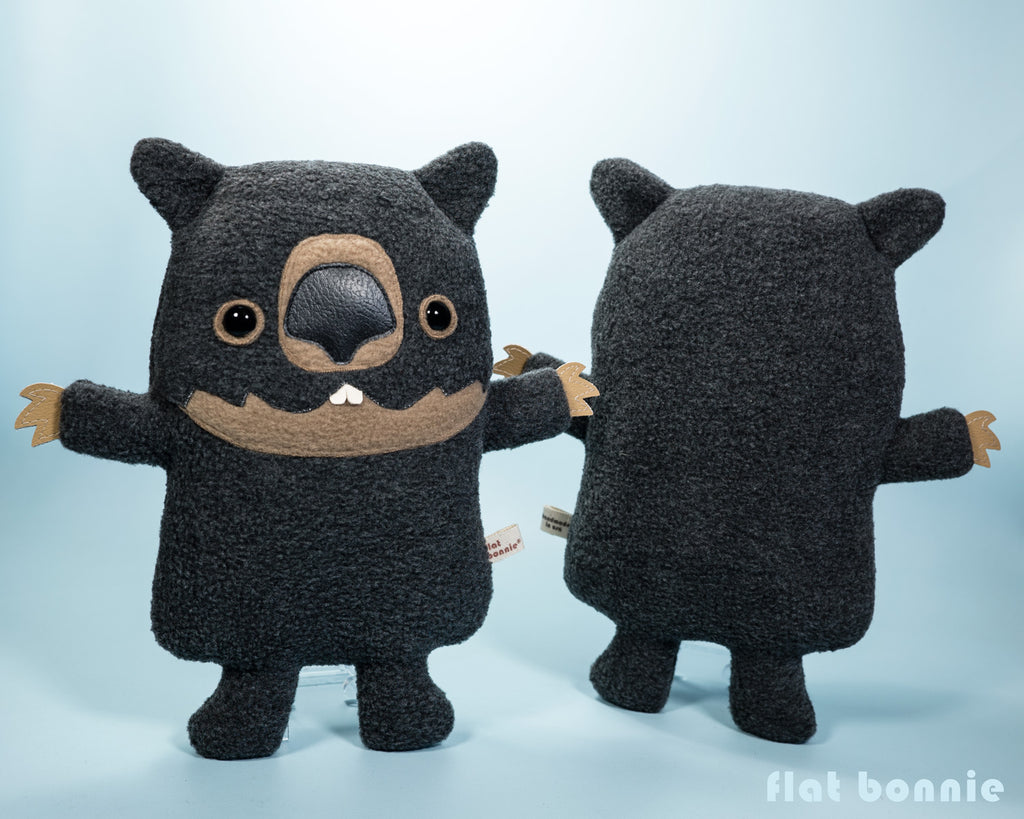This photograph displays a stuffed animal figure from both the front and back, side by side against a light blue background. The left side reveals the front of the stuffed animal, showcasing its detailed facial features and limbs, while the right side reveals its featureless back. The stuffed animal has a dark gray charcoal body, resembling a beaver with influences from Maurice Sendak's "Where the Wild Things Are" in its design. Its face features a distinctive black nose made of a different material, black eyes encircled by tan rings, and a tan mouth with two prominent white buck teeth protruding from the top. The ears are pointed and triangular, matching the beaver-like aesthetic. The snout and hands, each consisting of three pointed fingers, are also tan, contrasting the otherwise dark body. Additionally, a white tag with red writing is attached to the side of the figure. In the bottom right corner of the image, the words "Flat Bonnie" are displayed in white font.